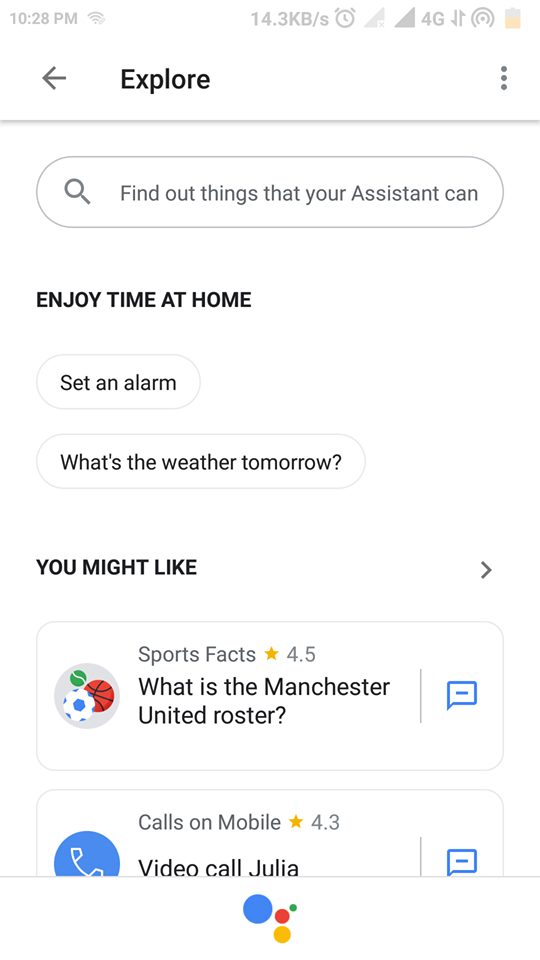This screenshot is taken from a mobile phone display, capturing several interface elements at 10:28 PM. The upper left corner displays the time, Wi-Fi signal strength, a data transfer rate of 14.3 kbps, and greyed-out phone signal indicators accompanied by a 4G icon. At the top, a grey horizontal line separates the header from the main content. The header features the word "Explore" along with a back arrow on the left and three vertical dots on the right.

Below the header, there's a search box prompting, "Find out things that your assistant can." Directly underneath, a prompt reads "Enjoy time at home" followed by a rectangular button with the text "Set an Alarm." Next, another curved-edged rectangle asks, "What is the weather tomorrow?"

Further down, the section titled "You might like" is indicated with a forward arrow on the right. Within this section, two rectangular cards with curved edges are visible, though the bottom of the second card is cut off. The first card is titled "Sports Facts" with a rating of 4.5 stars and the query "What is the Manchester United roster?" It features an icon on the left side—a circle containing three footballs colored green, red, and white with blue patches—and a blue-outlined speech bubble to its right. 

The second card is labeled "Calls on Mobile" with a rating of 4.3 stars and includes an icon of a white phone inside a blue circle on the left and another speech bubble to its right.

At the bottom center of the screen, a collection of colored circles is visible: a large blue circle, a smaller red circle, a smaller yellow circle, and a smaller possibly black or dark blue circle to the right.